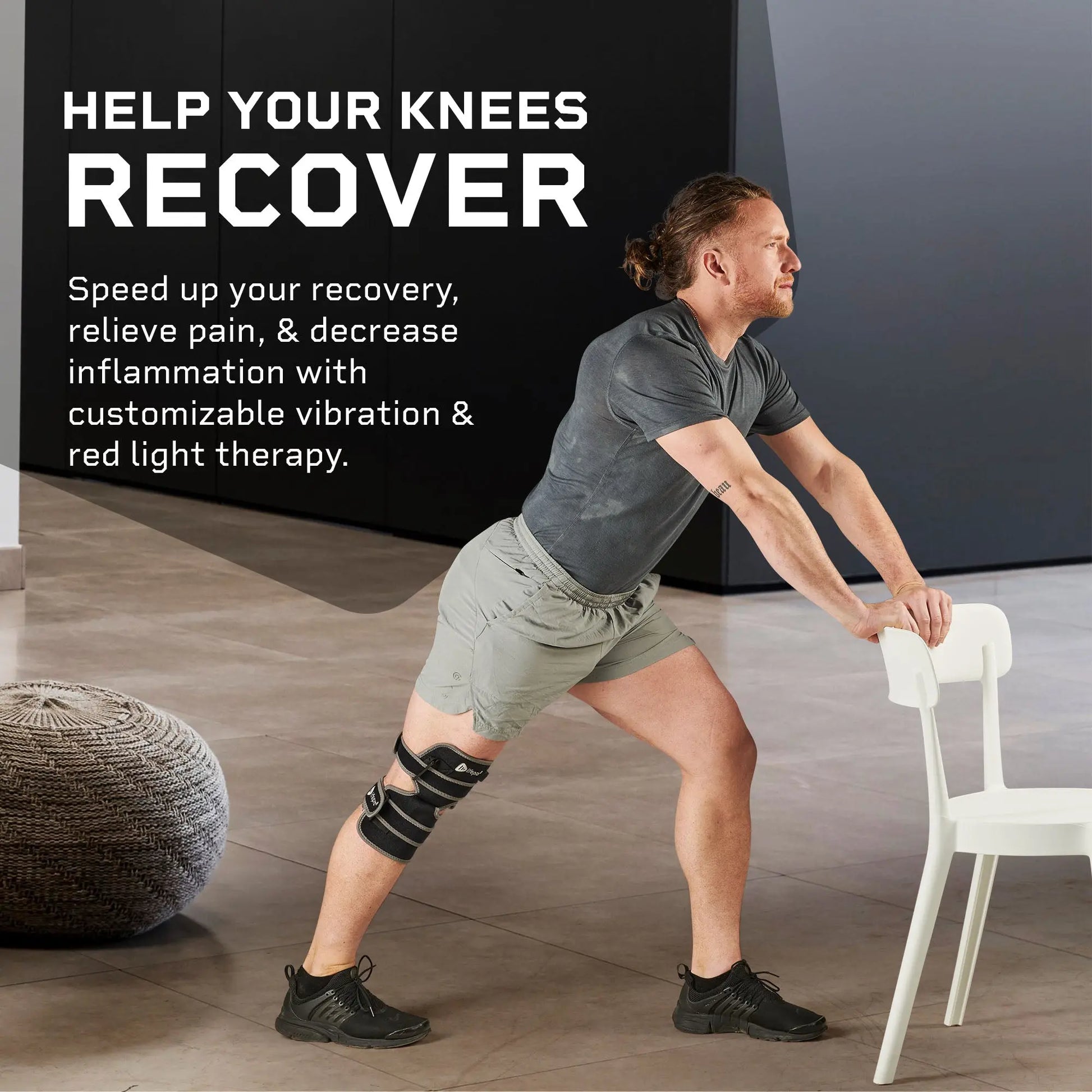This advertisement showcases an exercise device designed for physical therapy, featuring a fit, Caucasian man performing a stretching exercise. The man, with orange hair tied in a man bun and a subtle beard, is dressed in a short-sleeved, slightly dirty gray shirt, and light gray athletic shorts. He stands in an open room with a black wall in the background and a tiled floor below, using a small white chair for support as he leans forward, extending his body. His right leg is straight, bearing a black knee brace that covers both his knee and thigh, while his left leg is bent. To the lower right of the image, there's a mesh ball on the ground, adding to the physical therapy ambiance. Overlaying the scene, bold white text on the blackish gray background reads: "Help your knees recover. Speed up your recovery. Relieve pain and decrease inflammation with customizable vibration and red light therapy."